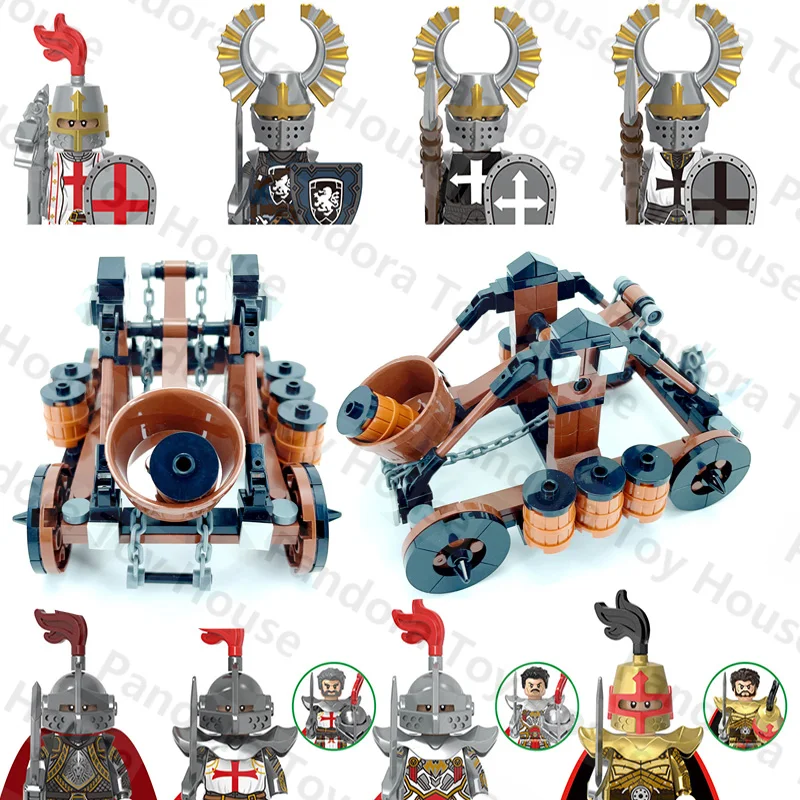This color photograph offers a detailed display of various medieval-themed building block toys, similar to Lego. The scene is set against a white background with a gray watermark that reads "Toy House." The arrangement features three rows of elements, with action figures and a central focus on a catapult.

At the top, four knights from a unified faction are pictured in front-view portraits, shown from the waist up. These knights wear diverse armor and headdresses adorned with feathers. The leftmost knight sports a silver helmet with a red feather and a Knight's Templar tunic marked by an orange cross, matching his silver shield. The knights to his right exhibit different military gear, featuring horns or bristles on their helmets and bearing lances with various insignias—one with a lion and others with white and black crosses.

The middle section showcases two views of a plastic catapult designed to mimic wood, complete with black wheels and a bucket mechanism. One image displays the rear view, resembling a small wagon with barrels attached and a missile set to launch. The side profile is oriented at a 45-degree angle, giving a clearer view of the catapult's mechanics.

The bottom row mirrors the top, depicting four more knights adorned in diverse armor. These figures also feature feathered helmets, with variations in their armor. The leftmost knight wears a red cape with gold and silver accents, while the next knight follows the Knight's Templar motif with a breastplate. Their counterparts include a knight with a golden bat insignia and another in bright gold armor, featuring a distinct helmet with a narrow eye slit and red arrow detailing akin to Nickelodeon's Avatar.

Overall, the image captures an intricate tableau of medieval action figures and weaponry, each with unique characteristics and detailed designs, framed as a cohesive and dynamic display.